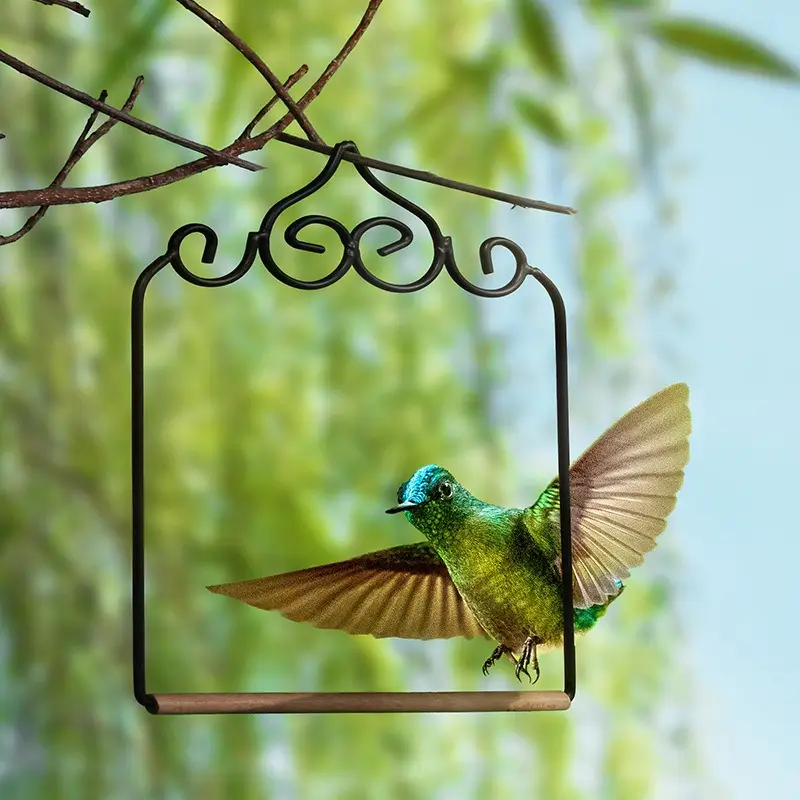In this outdoor photograph, a vividly green hummingbird, adorned with blue-green head feathers and a yellowish breast, is captured mid-flight with its wings wide open, showcasing their brown hue. The bird is about to land on a small metal swing with a wooden perch, which is suspended from a brown, twig-like tree branch. The background features a blurred scene of additional tree branches against a light green foliage and a blue sky, emphasizing the hummingbird as the central focus of the image. The bird’s large, expressive eyes add a touch of whimsy to the overall composition. It appears to be a digitally created image, given the bird’s strikingly vibrant colors and detailed features.